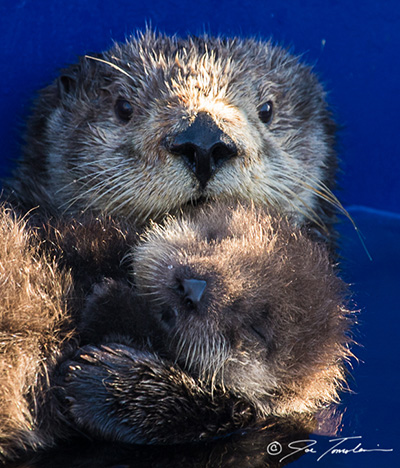This vertical rectangular image features a close-up of two sea otters against a dark blue background, seemingly cradling each other. The adult otter, speculated to be the mother, is larger with predominantly gray and white fur on its head and brown fur on its body. Its ears are back, almost hidden, and it has a glossy, black diamond-shaped nose, expressive black eyes, and long, white whiskers fanning out on either side of its snout. The baby otter, nestled affectionately against the adult, has softer, chubbier features with brown fur and white markings on its chin. Its tiny, brown paws appear to be under its chin or gently touching the mother. The sunlight casts a gentle sheen on their fur, highlighting the glossiness of their noses and the reflective quality of the adult otter's eyes. This heartwarming image also includes a small, cursive copyright symbol in the bottom right-hand corner.